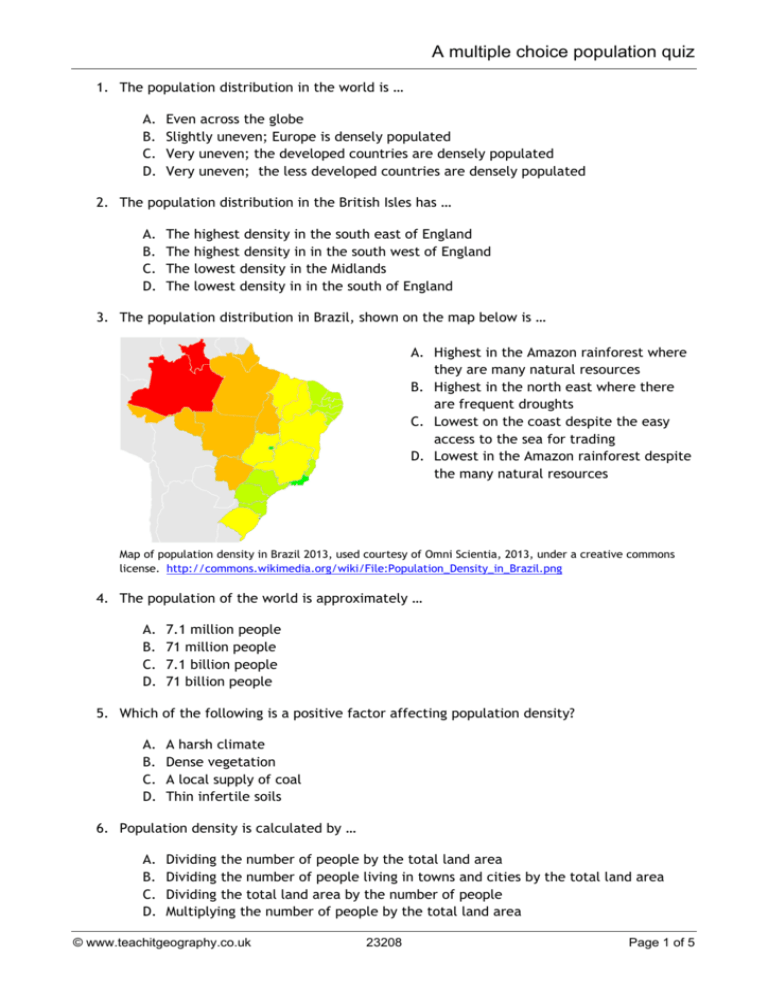**Detailed Caption:**

This image is a screenshot of a multiple-choice test on population geography, sourced from www.teachitgeography.co.uk. The test header reads "Multiple-Choice Population Quiz," and is followed by a horizontal line break. The page, numbered as "Page 1 of 5," contains six multiple-choice questions, each providing four options labeled A, B, C, and D.

1. **Population Distribution in the World:**
   The first question asks about the global distribution of the population, with options ranging from "evenly distributed across the globe" to "very unevenly distributed."
   
2. **Population Distribution in the British Isles:**
   The second question pertains to population density in the British Isles, with choices depicting various scenarios from "highest density in the south of England" to "lowest density in the south of England."

3. **South America Map (Question Includes an Image):**
   This question includes a map highlighting regions in South America, colored in red, orange, yellow, green, and dark green. It presents options related to population distribution, with highlights on areas such as the Amazon rainforest and the presence of natural resources. The map is referenced from Wikipedia, with a link provided.

4. **World Population Estimate:**
   The fourth question requests the approximate population of the world, with answer choices distinguishing between millions and billions of people.

5. **Positive Factors Affecting Population Density:**
   The fifth question asks which of the provided options is a positive factor that affects population density.

6. **Calculation of Population Density:**
   The final question inquires about the method used to calculate population density. 

The bottom footer below another horizontal line break includes copyright details, the website (www.teachitgeography.co.uk), and the document number 23208.